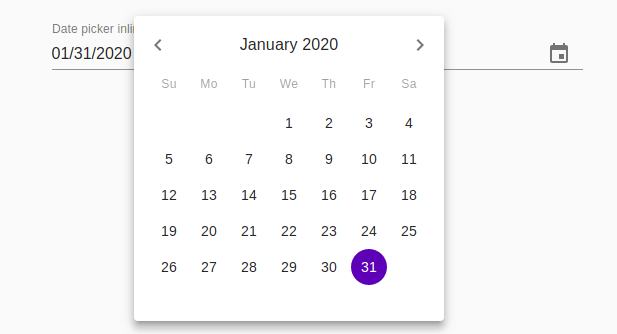A close-up screen capture of a digital interface displays a date picker. In the background, "January 31, 2020" is clearly visible, while a prominent pop-up window in the foreground shows the calendar for January 2020. The calendar includes navigation arrows on either side, allowing users to navigate through different months. The selected date, January 31st, is encircled in blue, indicating it is a Friday. This interface appears to be for scheduling purposes or setting a date on a device, although its exact function isn't specified.